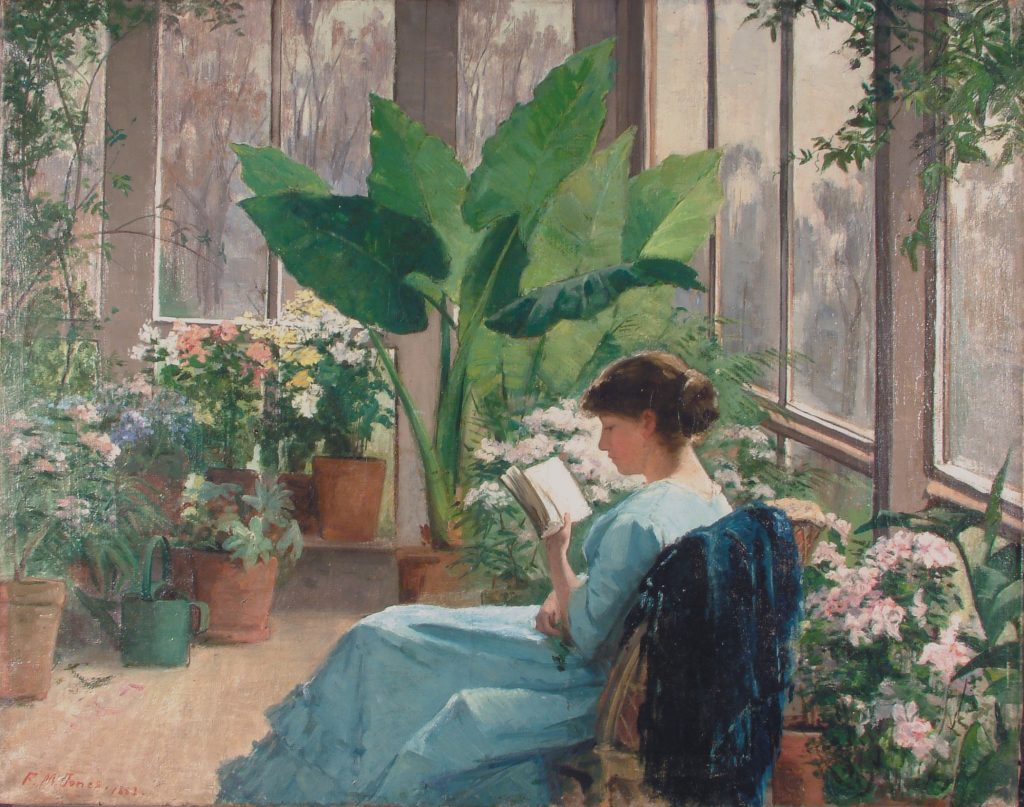This detailed painting depicts a young woman, dressed in a long sky blue dress, sitting in a brown wicker chair with a dark blue blanket draped over its back. Her brown hair is pulled up in a bun, and she is engrossed in reading an open book with white pages. Central in the composition, she is situated at the bottom middle of the image. The setting is lush and vibrant, filled with various plants and flowers. A large plant with big leaves occupies a corner, while white flowers with green leaves are positioned behind and beside her. Pink, blue, darker pink, yellow, and white flowers with green foliage are scattered around, and hanging plants are seen in the top right and left corners. The room features floor-to-ceiling windows framed in gray or white, offering a view of red or orange trees with green hanging elements and brown branches outside. The floor of the room is light brown wood, adding warmth to the scene. The two walls behind and around her are lined with numerous potted plants, creating a serene, garden-like atmosphere. A signature, presumably by the artist F.M. Jones, is visible on the painting.